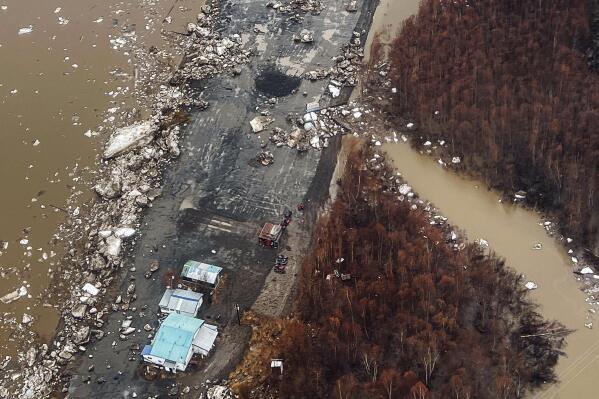This aerial photograph captures the aftermath of what appears to be a natural disaster, possibly a storm. Central to the image is a narrow gray ground area intersected by a long, debris-laden highway. Scattered across this ground are several houses surrounded by considerable fallen debris, suggesting significant destruction. 

To the left of the ground area lies a muddy, brown-colored body of water, similarly filled with debris, including rocks and stones along its edges. On the right side, a narrow stream, also carrying brown water, cuts through a dense cluster of trees. These trees, notably brown and red in color, could indicate either a seasonal change, such as late fall, or damage from a forest fire. 

A striking element within the devastation is a small, blue building surrounded by pavement, standing amidst the debris and fallen trees. The aerial shot, likely taken from a drone, vividly shows the polluted water gradually merging into a larger river, encapsulated by a triangular section of brown and barren trees on one side and a larger swath of similarly affected trees on the other. This image poignantly visualizes the chaos and disruption caused by the disaster.